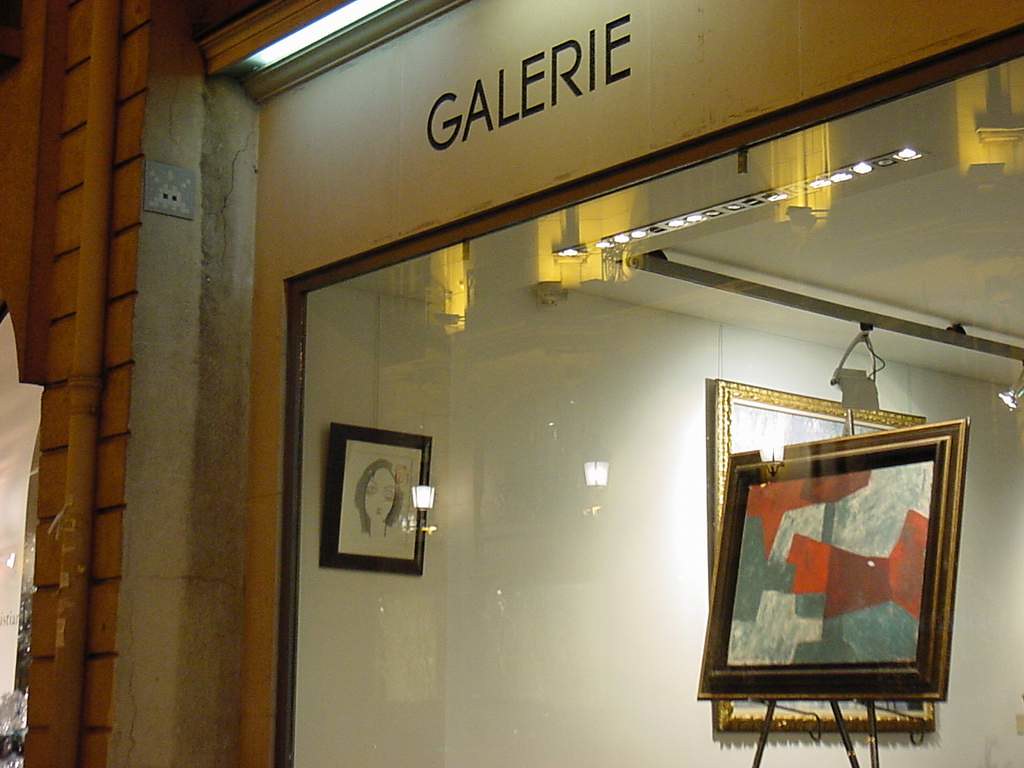This detailed photograph shows the exterior of an art gallery at night or dusk. The storefront is distinguished by a large pane glass window, framed by a brick wall surrounding it and an orange-reddish tiled section with gray accents. Above the window, in black stenciled letters, the word "GALERIE" is spelled out, illuminated by a fluorescent light, and bordered by what appears to be a gold-colored material. 

The interior of the gallery, visible through the window, features a minimalist display with white walls and sparse art pieces. Track lighting highlights the artwork inside, including a prominent standalone framed piece directly facing the window. This piece, in a black frame, depicts a stylistically rendered woman's face, seemingly drawn in pencil. Additionally, another framed artwork, set in a bronze frame and displaying geometric shapes in red, blue, and gray, also draws attention. The left side of the image reveals a brown paneled wooden wall and a vertical cement pole, adding texture to the composition. Further left, a reflective sign and a pixelated sun-like tile design enhance the scene, completing the visual narrative of the storefront art gallery.